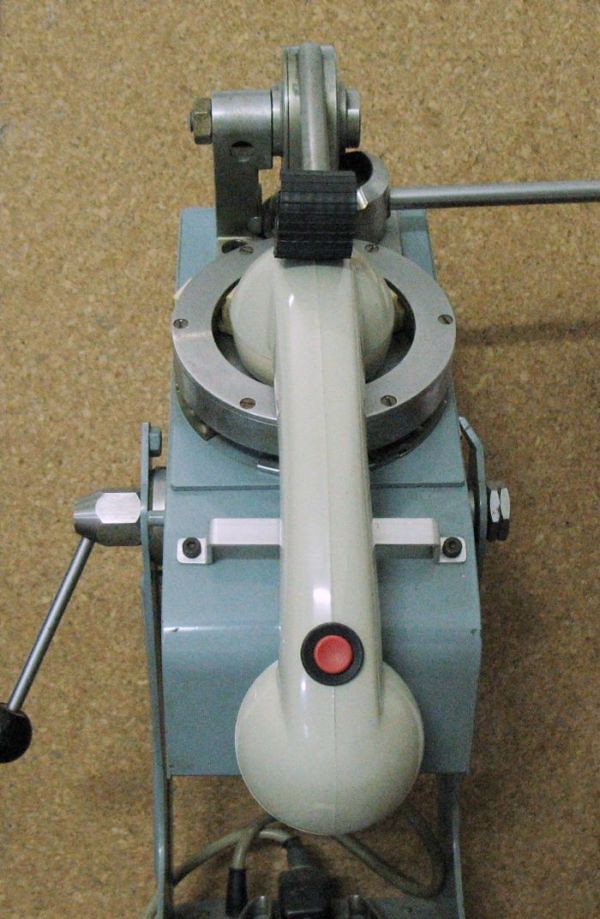The image depicts a complex metallic device set against a tannish-brown background that resembles plywood or laminate flooring. The apparatus features a slender, rectangular body with a drab bluish-green coloration. At the top, there's a vintage-style telephone receiver, light gray to off-white in color, mounted horizontally. This receiver includes a red button on its underside and is held in place by circular metal holders at both ends, with a black rubber stopper on one end.

To the left side of the device when facing it head-on, there's a handle with a large black knob, seemingly designed for twisting or tightening. A silver dial protrudes from the right side (visually left when viewed head-on), ending in a black circular handle. Additionally, a pipe and other metallic components extend to the right and top of the device.

Wires are visible at the bottom, hinting at its electrical nature. A foam pad rests on a metal bar that sticks up from the structure, and a small screw is noticeable on one side. The entire setup suggests an intricate contraption, potentially a specialized tool or machine.